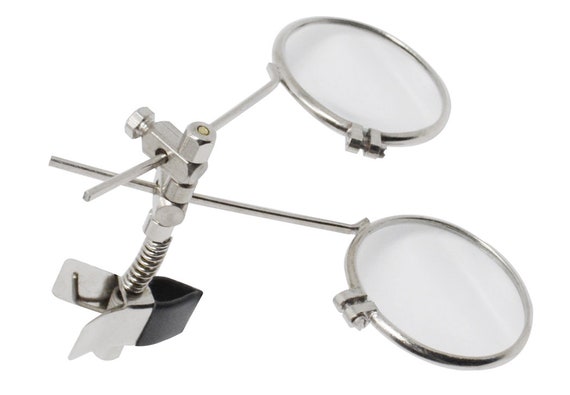This photograph displays a metallic contraption set against a completely white background, which could be indicative of post-editing to eliminate shadows. The device features a clamp at the bottom, composed of silver and black materials, potentially black plastic or rubber. This clamp allows the contraption to be securely attached to various surfaces. Extending from the clamp is a slender metallic rod adorned with bolts and nuts, holding two eyeglass-shaped pieces. These eyeglass pieces, with silver edges and white centers, appear to be adjustable and capable of independent movement, akin to a jeweler's loupe. The apparatus may serve functions in precision tasks, such as in an eye doctor's office for examination or for providing magnification.